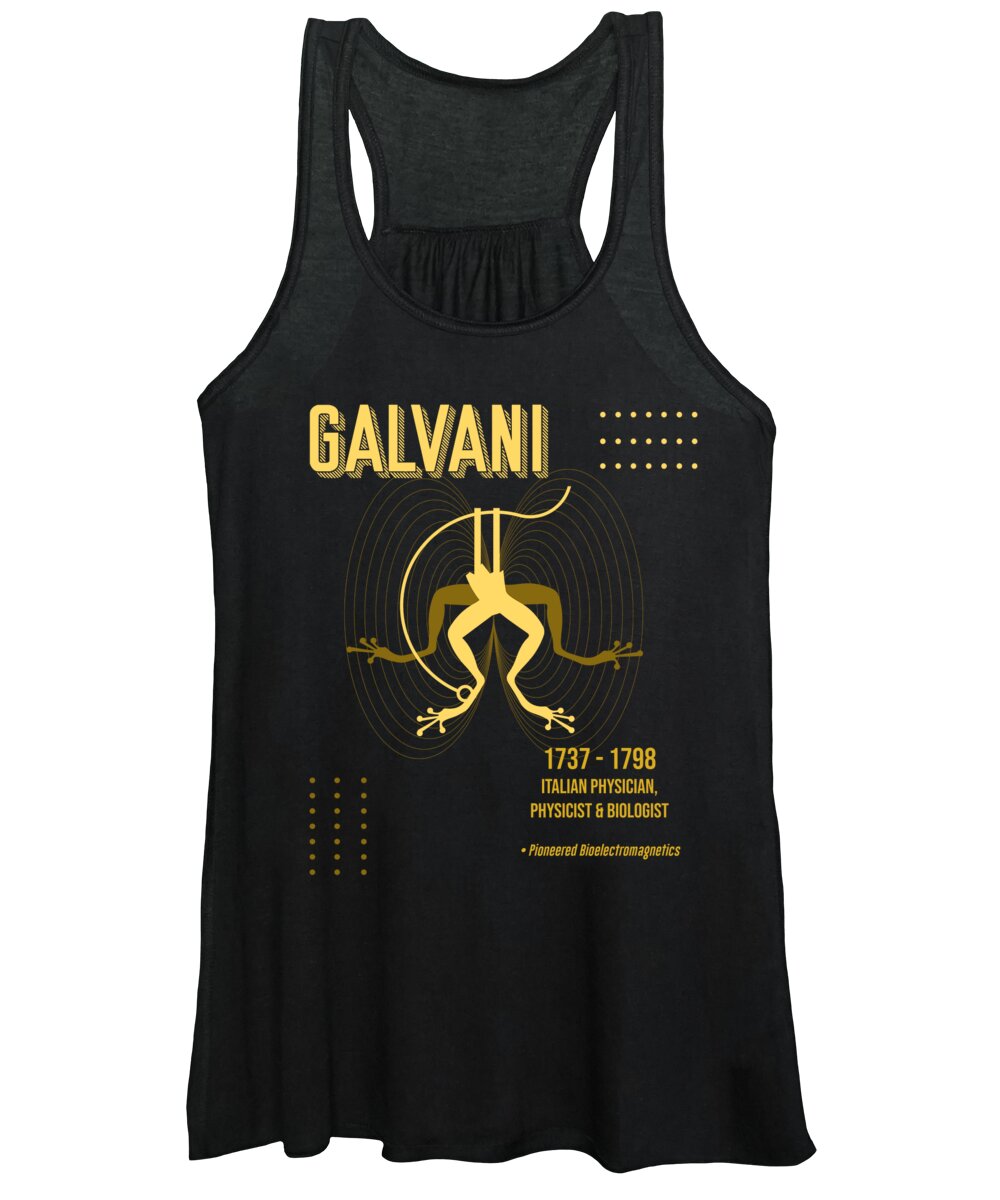The image showcases a black women's tank top displayed against a pure white background. Dominating the upper middle section of the tank top, the word "Galvani" is prominently printed in bold yellow letters. Below this, an intricate graphic features two pairs of frog legs in different shades of yellow: a lighter pair overlays a darker pair, forming a mirrored spiral pattern with an expanding ellipsis shape. Between the legs, multiple circles create a concentric design, giving a dynamic visual effect. Adjacent to this image is golden text that reads "1737 to 1798" followed by "Italian physician, physicist, and biologist," highlighting Galvani’s pioneering work in bioelectromagnetics. Additionally, three horizontal lines of light yellow dots are positioned near the top right, while three vertical lines of similar dots adorn the bottom left corner, further enriching the tank top's design elements.